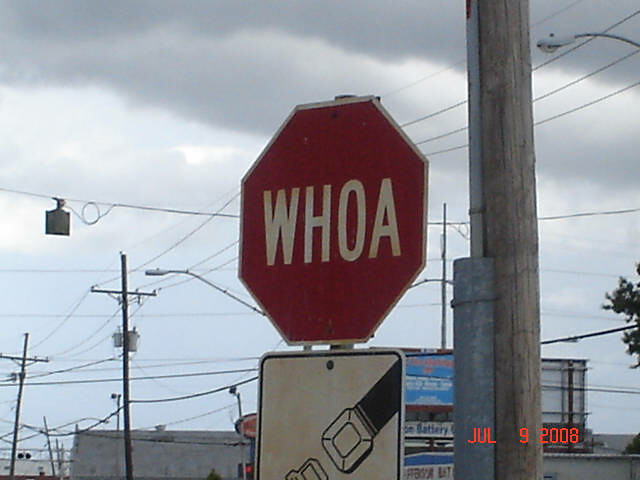The image, captured with an upward angle, predominantly features a gray, heavily overcast sky, contributing a moody, somber tone. A time stamp in red, located at the bottom right corner, specifies the date as July 9, 2008. Dominating the right side of the frame is a large wooden pole, likely a utility or lighting pole. To its left, the upper portion of a unique street sign is visible. Congruent with a standard stop sign in its octagonal shape, white border, and red background, this sign humorously displays the word "WHOA" in white letters. Positioned just below it, partially visible, is another street sign, either square or rectangular, featuring a white background with a black border. From the upper right segment of this second sign, a portion of a seat belt intrudes into the frame, emphasizing an unexpected, whimsical touch in the otherwise mundane street scene.